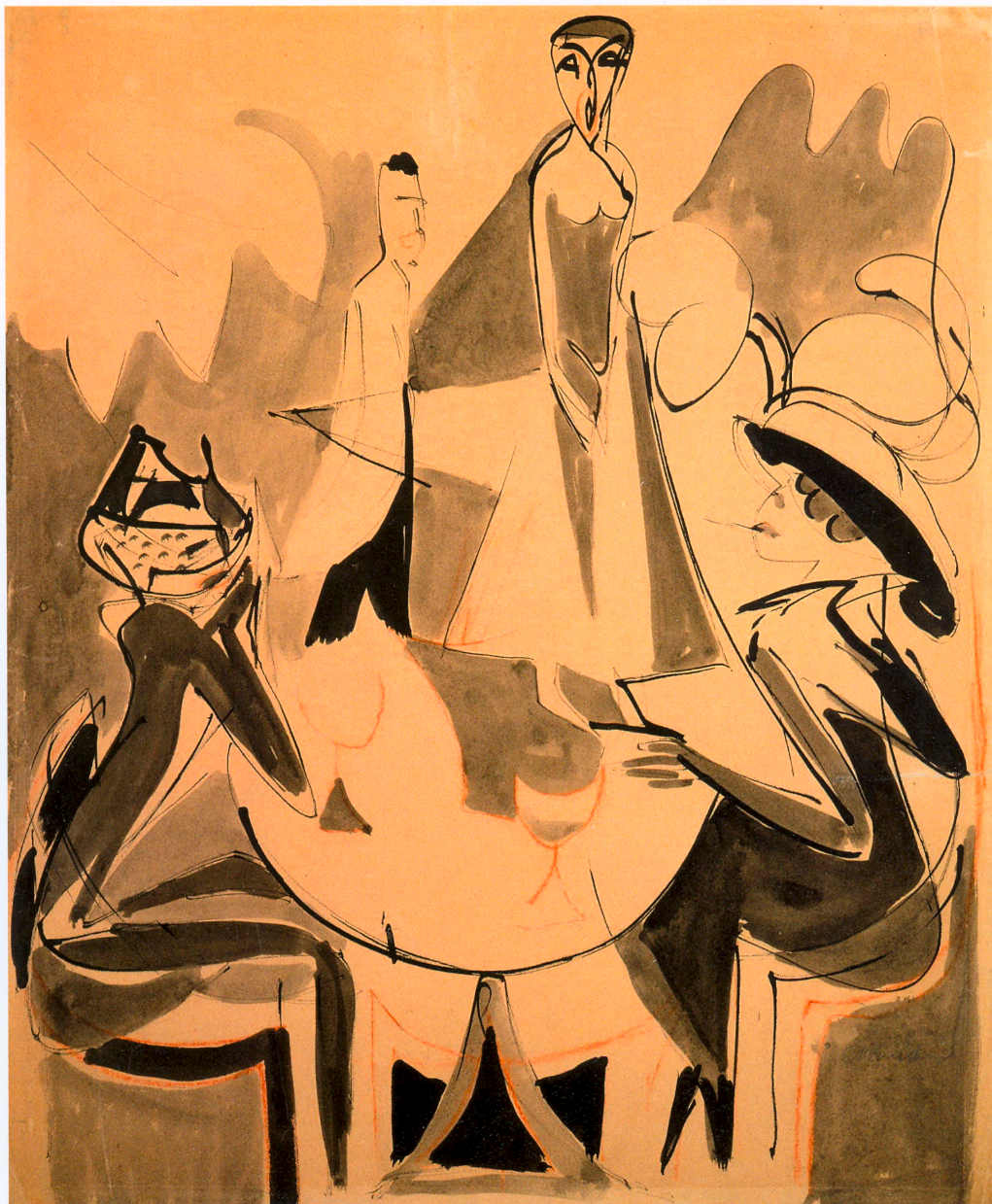This vibrant, esoteric modern artwork is reminiscent of the 1980s style with its predominant peach-orange background. The piece, seemingly created with a combination of ink, markers, and possibly watercolor, features a sketch-like texture. Central to the composition is a black and gray outlined table, upon which sit two elegantly dressed women in evening attire, complete with dresses and hats. The woman on the right is engrossed in a menu, a cigarette in her mouth, and her legs folded beneath the table. She wears a tall hat from which some of her hair peeks out, accentuating her pointed chin. Opposite her, the second woman, donning a slightly shorter hat, appears to be gazing attentively at a surprised-looking woman standing in the background. This standing figure, positioned at the top of the vertically aligned piece, has short brown hair and a distinctive diamond-shaped mouth forming an 'O', suggesting surprise. Dressed in a gown, she seems to be engaged in the scene. Behind her, a man, possibly a waiter in a long white coat and black pants, walks by in the further background. The overall composition highlights a blend of surreal, abstract features with intricate social interactions, all bathed in the striking orange hue.